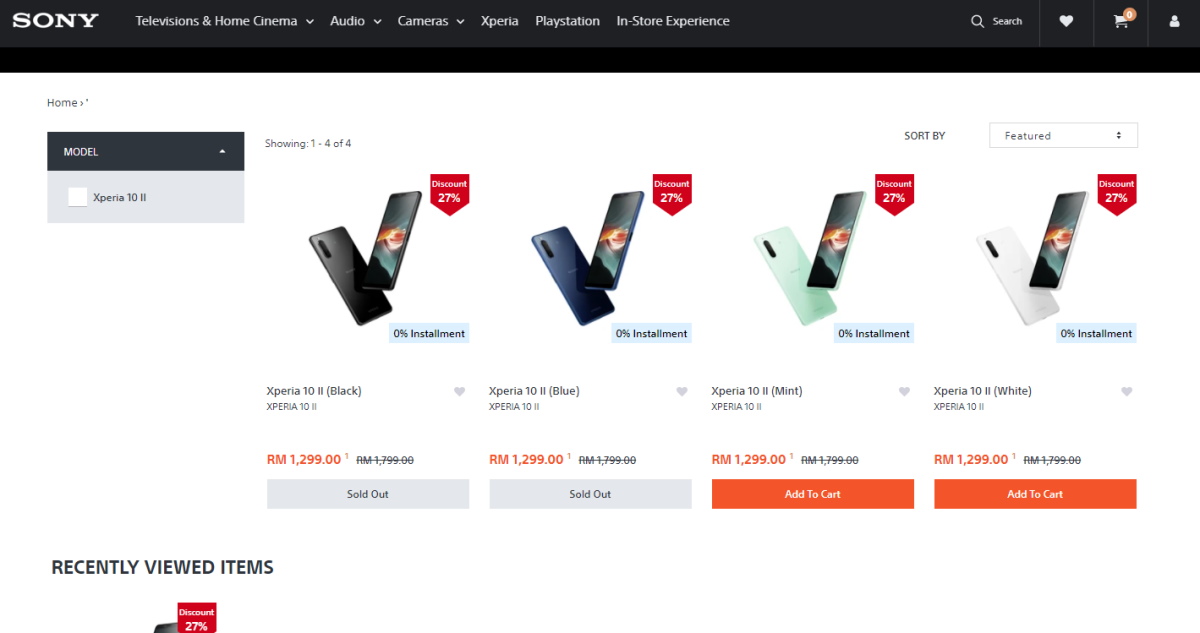This is a detailed and cleaned-up caption for the given screenshot description:

---

The screenshot captures the upper section of a Sony website, excluding the browser borders. A prominent black banner spans across the top, with "Sony" displayed in the upper right corner. Directly below, a series of navigation tabs are visible, including categories such as "Televisions & Home Cinema," "Audio," "Cameras," "PlayStation," and "In-Store Experience," each featuring drop-down menus for further options. On the far right side of the banner, icons for search, favorites (heart), shopping cart, and user avatar are lined up.

Beneath the navigation bar, four Sony Xperia phones are showcased side by side, each showing a discount of 28% highlighted in red. The prices for all four phones are listed as RM 1299. The first two phones on the left display a gray bar at the bottom, indicating they are sold out. In contrast, the two phones on the right have an orange "Add to Cart" button beneath them.

In the lower-left section of the screenshot, there's a "Recently Viewed Items" text label. Partially visible beneath this is another item, showing a discount of 27% in red, but most of the details are cut off.